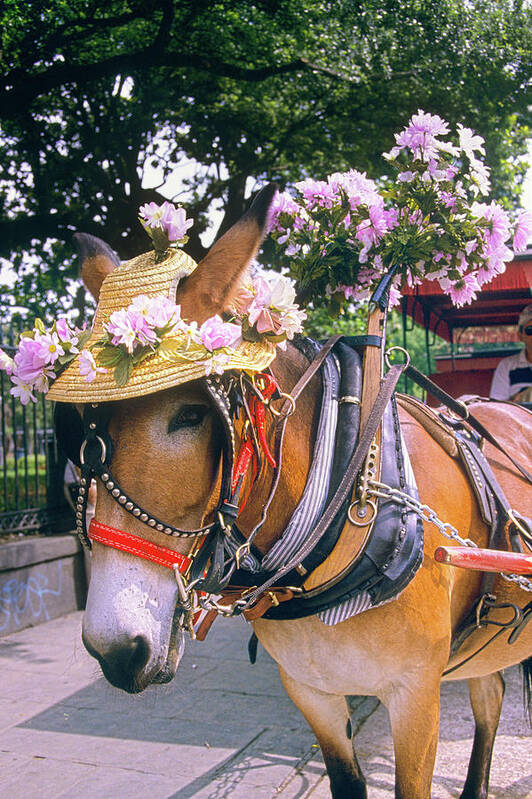This photograph features a close-up of a brown donkey adorned with a straw hat that has holes for its ears to protrude through. The hat is decorated with a wreath of pink and light-colored flowers on the brim. The donkey also wears a large bridle and a heavily laden saddle, suggesting it is harnessed to a cart or carriage, barely visible in the background. Its white muzzle contrasts with its dark, almost black, lower legs. The setting appears to be near a sidewalk adjacent to a park, marked by an iron fence on one side. Only half of a person is seen beside the donkey, which looks straight ahead, standing on a road or path.